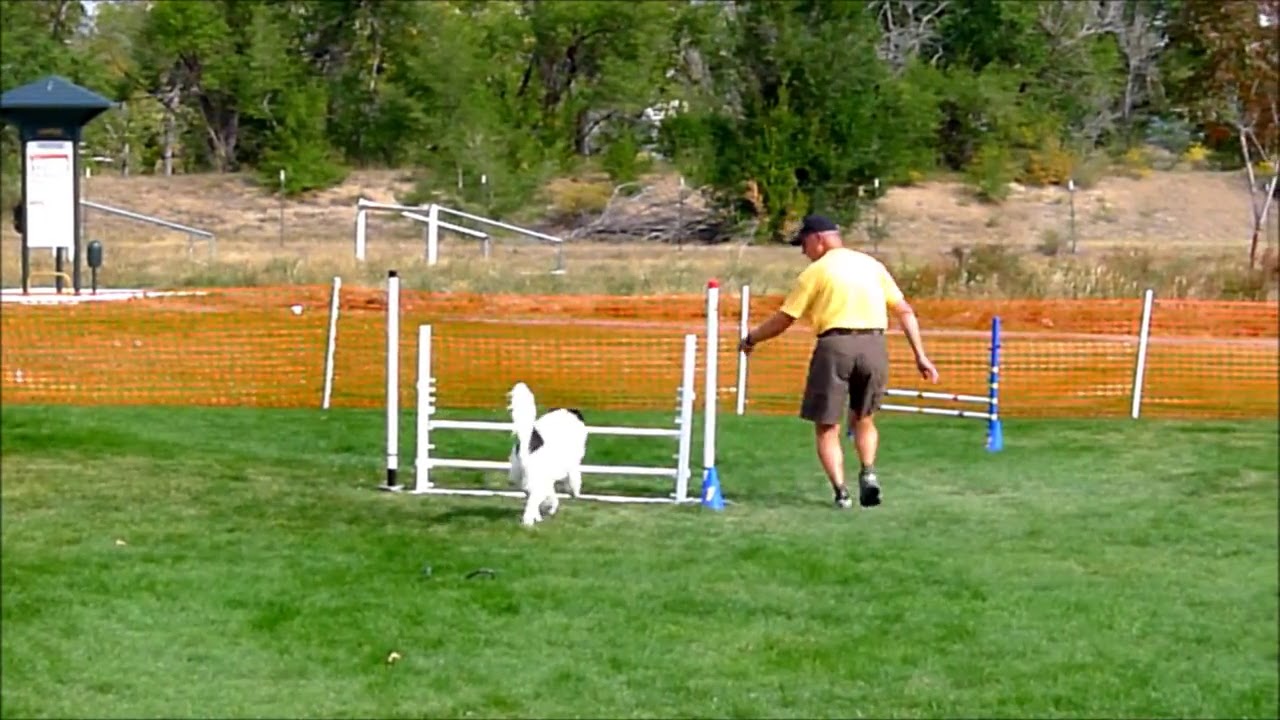In this detailed park scene, a grassy field stretches across the lower part of the image, flanked by an orange plastic safety fence in the background. In front of the fence, a series of white poles, arranged for dog agility training, stand out prominently. Centered in the image, a white dog with black ears and a black-tipped tail appears to be mid-leap over one of these white pole obstacles, its front legs thrusting forward in anticipation.

To the right of the dog stands an older Caucasian man, caught in motion as he likely guides or encourages his dog. The man, facing the same direction as the dog, is wearing a yellow t-shirt tucked into dark gray shorts, a dark navy blue baseball cap, and running shoes. Over his shoulder, the strap of a visible bag hangs. Directly in front of him and the dog is a white agility jump with two bars that the dog is presumably training to clear.

This active scene is set against a backdrop where the fenced-off grassy training area transitions into a dirt hill crowned with trees. Peaceful and focused, this image captures a moment of outdoor training and companionship between man and dog in a dedicated park area.